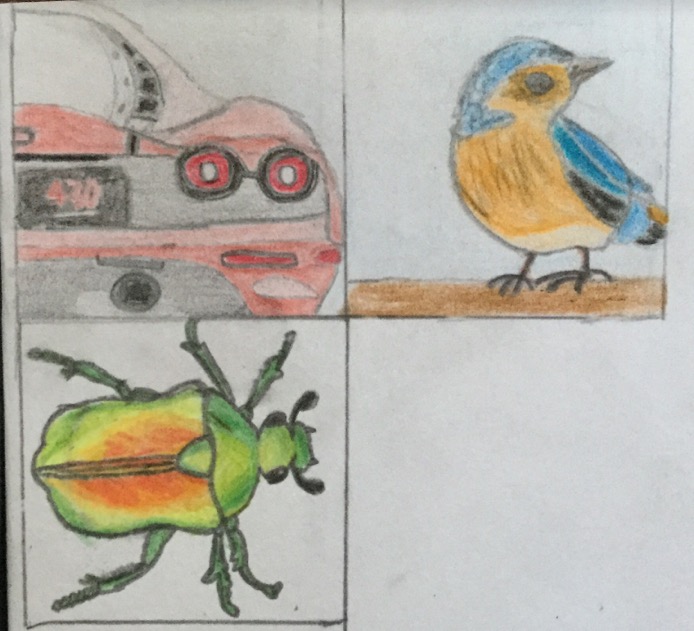The image consists of a white piece of textured and smudged paper sectioned into four quadrants: three of which contain colorful sketches, and one bottom right quadrant that remains blank. In the top left quadrant, there’s a detailed drawing of the rear end of a red sports car with a 430 license plate in red and black trim around red taillights. The car features a striking red body with a contrasting white roof. The adjacent top right quadrant depicts a perched bird on a brown branch, showcasing vibrant blue and yellow feathers with a white belly and face, and its head tilted to the right. The bottom left quadrant houses a depiction of a green beetle with three legs on each side, black antennae, and a complex color gradient on its back, moving from an orange center to yellow, and then to green. The paper, set against a dark background, bears noticeable black and gray smudges, adding depth and dimension to the overall presentation.